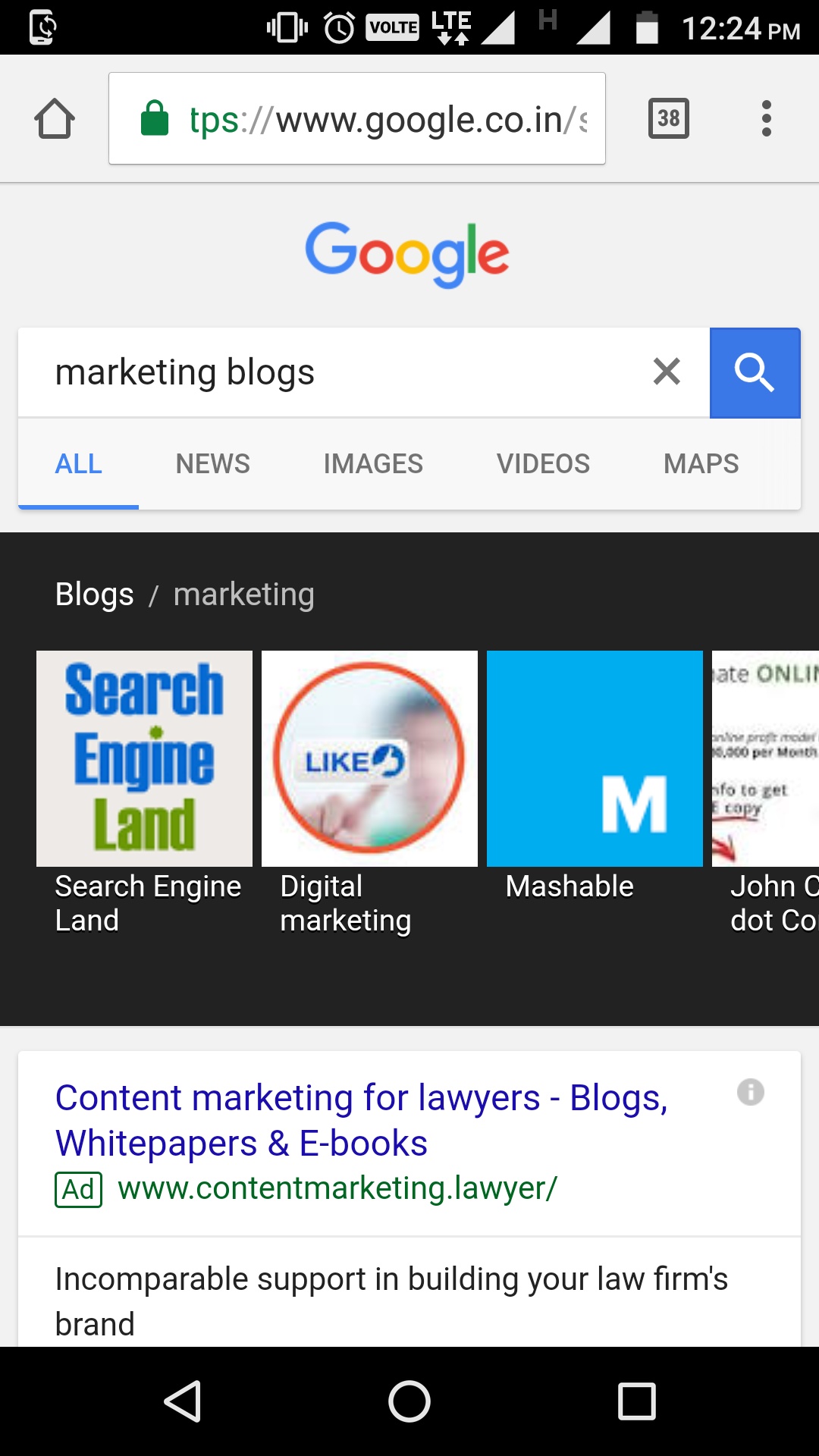Screenshot of a Google Search Results Page on a Mobile Device:

At the top of the screenshot, the URL bar displays "Google in India," accompanied by the Google logo just below it. The search query entered in the white search bar reads "marketing blogs." Below the search bar, there are five tabs for filtering results: "All," "News," "Images," "Videos," and "Maps." 

The search results begin with organic listings featuring prominent marketing blogs such as "Search Engine Land," "Digital Marketing," and "Mashable." Interspersed among these results, there are also sponsored ads. One notable ad displays the URL "www.contentmarketing.lawyer" in green text, indicating it is a paid advertisement. The accompanying ad text in black reads: "Incomparable support in building your law firm's brand," highlighting the focus on content marketing services for law firms, including blogs, white papers, and e-books.